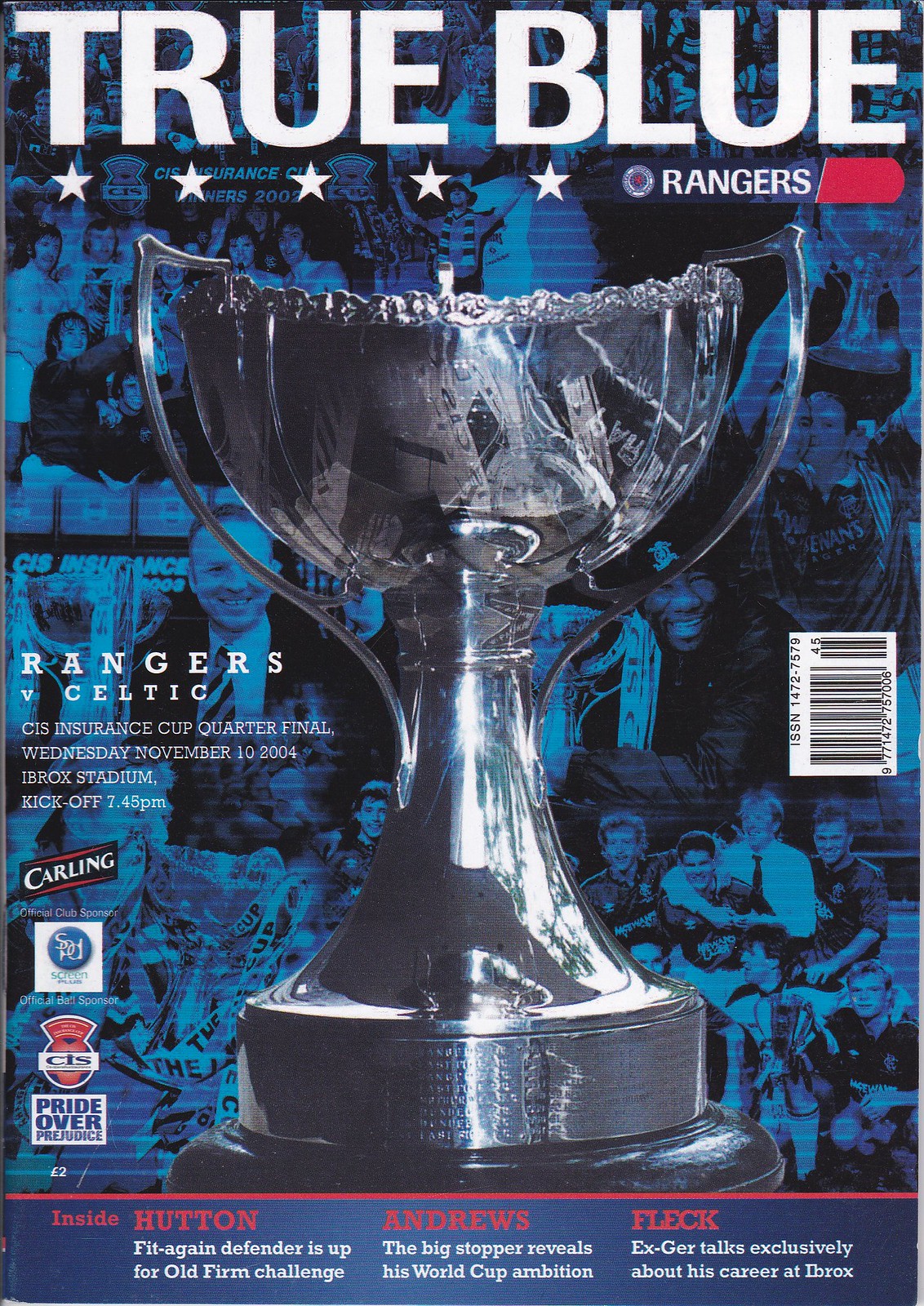The image is a magazine cover with the title "TRUE BLUE" prominently displayed at the top in large white text. Below the title are five small white stars. Next to these stars is the word "RANGERS," which is also accompanied by the Rangers sports team logo. Dominating the center of the cover is a large, reflective silver trophy cup. To the left of the trophy, white text reads "Rangers vs. Celtic, CIS Insurance Cup Quarterfinal, Wednesday, November 10, 2004, at Ibrox Stadium. Kickoff: 7:45 p.m." The background consists of a blue collage featuring pictures of fans in stadiums. On the left side, there are logos, including one for Carling, along with text that reads "PRIDE OVER PREJUDICE," while a black and white barcode is situated on the far right, turned sideways. At the bottom of the cover, a dark blue border includes text lines in red and white, with details like "Inside: Hutton, Andrews, Fleck" and "Fit again defenders up for the old firm challenge."